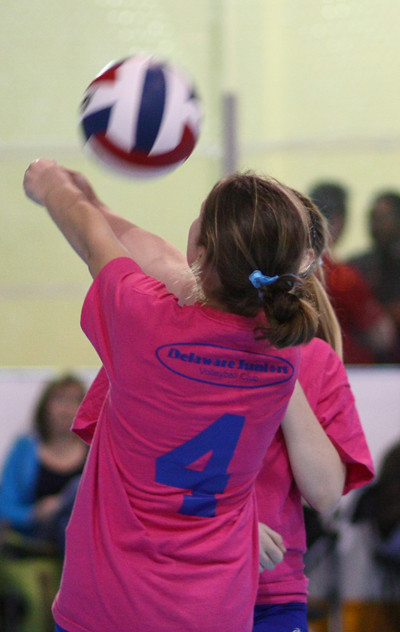In this photograph taken at a middle school or high school volleyball game, a Caucasian girl with brown hair is seen from the back, wearing a bright pink t-shirt. Her hair is tied in a ponytail adorned with a small blue bow. The shirt features a large blue number four printed on the back, above which is an oval insignia that reads "Delaware Juniors Volleyball Club," although the additional letters within the oval are indistinct. The girl is in the act of bumping a volleyball with her forearms, her hands clasped together. The volleyball is strikingly patterned with red, white, and blue stripes. In the out-of-focus background, blurred spectators are visible, while another girl, also Caucasian with brown hair in a ponytail and wearing a similar pink shirt, stands slightly behind her. The girl's face is not visible, maintaining the focus on her athletic posture and the dynamic movement of the game.